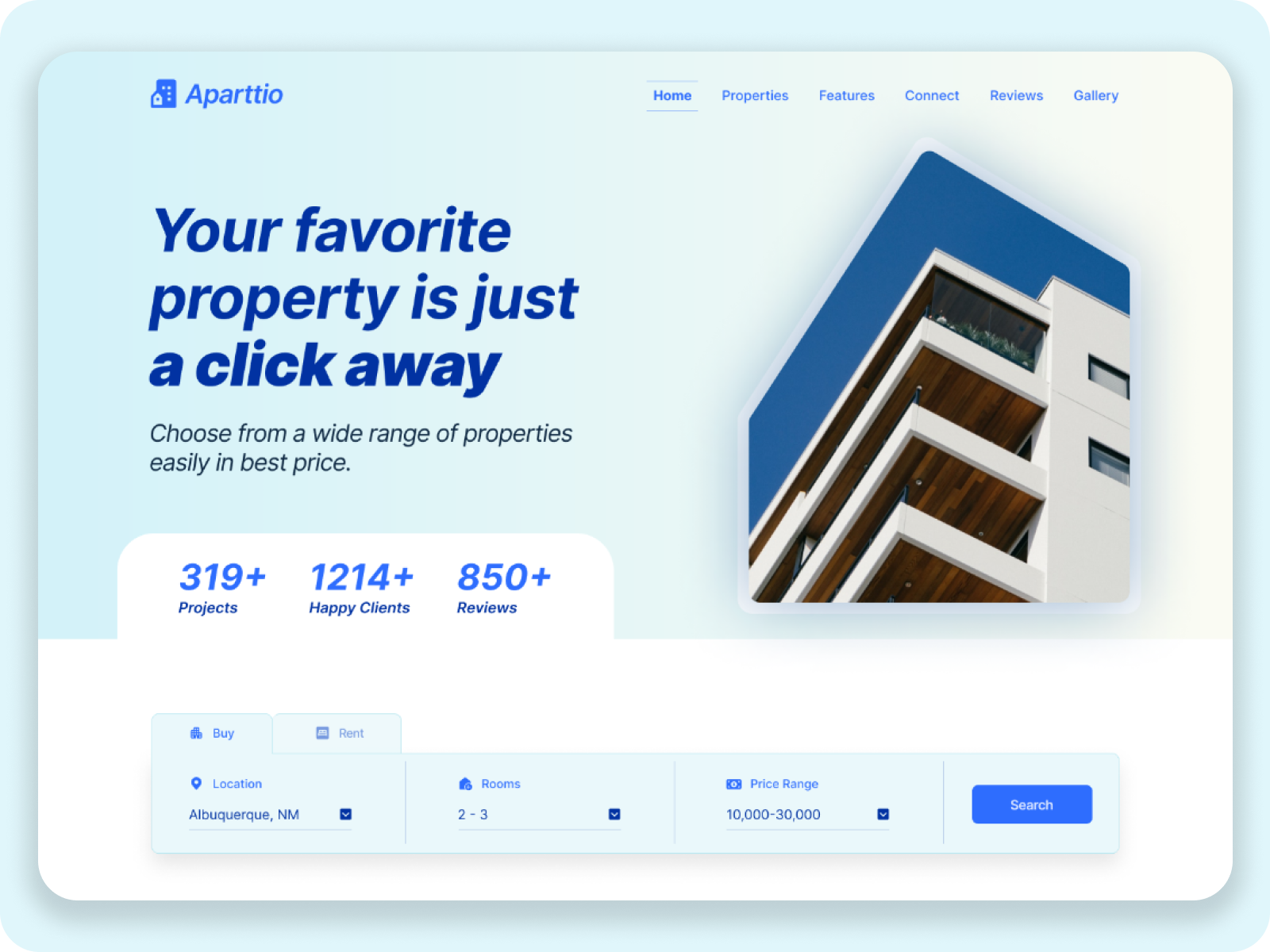A screenshot with a light blue background showcases the ParkTO website interface. The top navigation menu includes tabs labeled "Home," "Properties," "Features," "Connect," "Reviews," and "Gallery." Below this navigation bar, a striking image of a building is prominently displayed alongside a motivational tagline, "Your favorite property is just a click away." The website highlights the ease of choosing from a wide range of properties at the best prices. 

Key statistics presented include:
- 319+ projects
- 1,214+ happy clients
- 850+ reviews

The site offers options to "Buy" or "Rent" properties and features search filters for "Location" (such as "Faber-Kruge, NM"), "Rooms" (ranging from 2 to 3), and "Price Range" ($10,000 to $30,000). At the bottom of the search area, there is a blue rectangular button with the word "Search" in white text, inviting users to begin their property search.